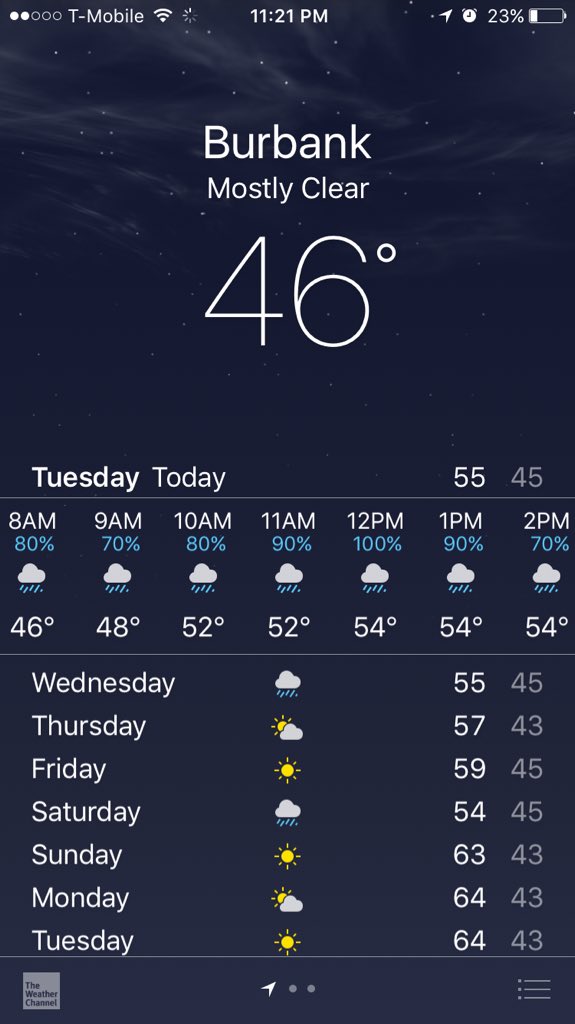The image depicts a detailed weather forecast provided by The Weather Channel. It spans from Sunday to Saturday, showing temperature predictions and weather conditions for each day. 

On Tuesday, the high is forecasted to be 55°F, with mostly clear skies. Thursday's forecast indicates clouds and cooler temperatures, also around 55°F. The weekly temperature range varies from 43°F to 63°F, depending on the day and time. Precipitation probabilities are also indicated throughout the week, with rain chances peaking at 80% around noon and 70% around 9 a.m. on Tuesday.

The user interface includes various icons and visual indicators, such as white and black dots, arrows pointing to the bottom right, and blue and white cloud symbols, representing different weather conditions and times. The forecast includes percentage chances of rain for specific times across the week, highlighting a detailed breakdown of anticipated weather patterns.